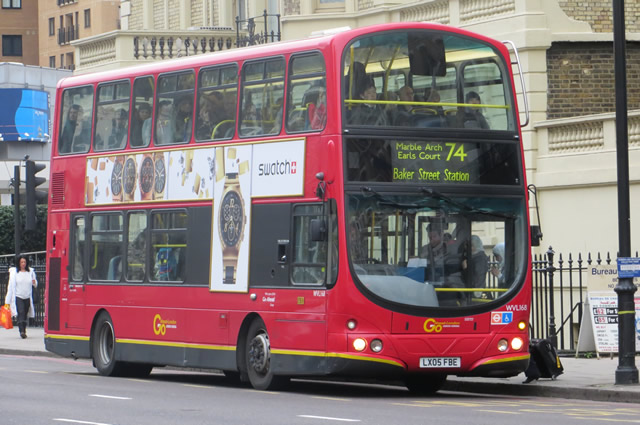This detailed photograph captures a vibrant red double-decker bus prominently positioned in a designated bus lane marked by yellow lines on a gray asphalt street, further distinguished by white dashed lines in other traffic lanes. The bus's digital marquee displays the route details: “Marble Arch, Earl's Court, 74, Baker Street Station.” The bus is notably packed with passengers visible through its glass windows, with the driver situated on the lower level and more passengers filling the upper deck. An eye-catching Swatch advertisement featuring multiple watch faces and the brand's iconic red and white cross logo spans the bus’s side. The bus, with its distinctive yellow and black lower border, bears the license plate LX05FBE. In the background, tall stone buildings in cream and brown hues frame the scene, adding to the urban ambiance. A woman in a white sweatshirt and black pants, holding an orange bag, walks behind the bus, while a tall utility pole stands to its right. Adding to the street's bustling atmosphere, a sandwich board sign with partially legible text reading “Bureau” is visible. This lively depiction evokes a classic downtown cityscape, likely in London.